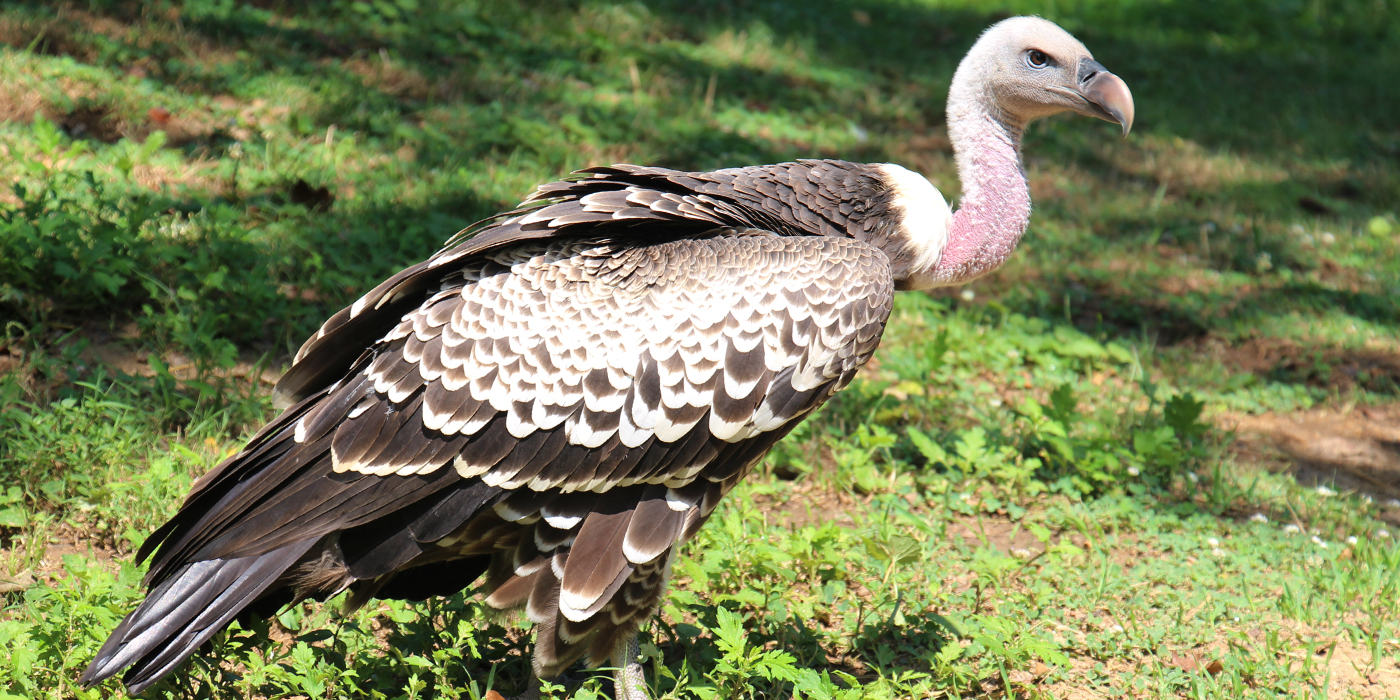In this detailed photograph, we see a close-up side profile of a bird, likely a vulture or buzzard, standing on the ground amidst green grass and scattered vegetation. The bird features a striking contrast of colors: its cottony white and black feathers cover its body, while its bald neck and face display a pinkish-white texture. The bird's head, whitish in hue, supports a sharp, curved beak that is a faded orange-brown. Its intense black eye is fixed to the right, giving an impression of focus or vigilance. The background, a field with a mix of weeds and some sand, is clear in the foreground but gradually blurs towards the back, highlighting the bird as the focal point. The setting, undoubtedly in nature, suggests an outdoor environment, perhaps a park or forest floor.